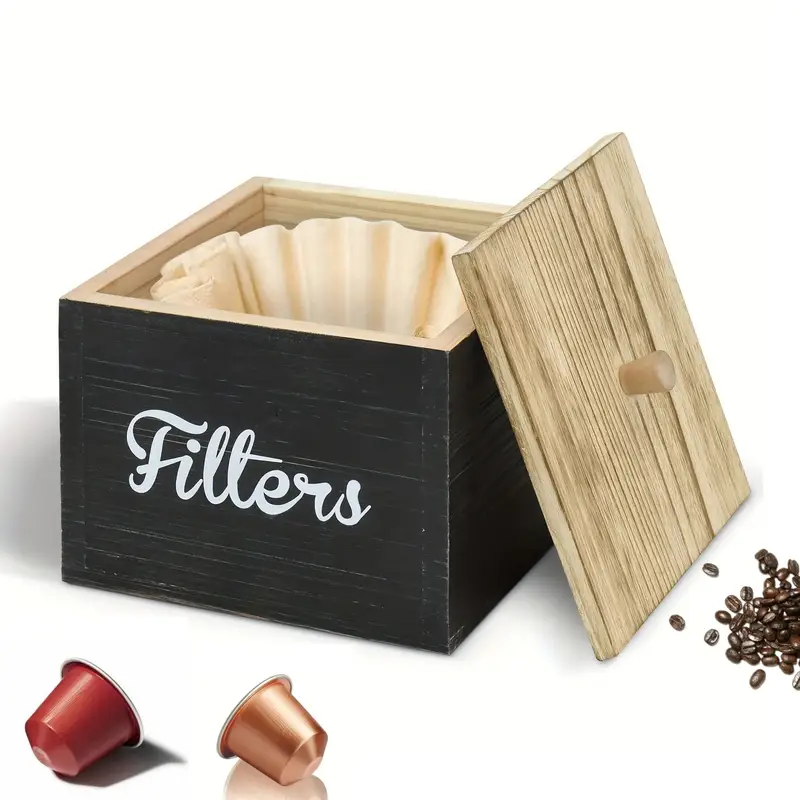This detailed illustration features a square wooden box designed to store coffee filters. The box, painted black on the exterior, prominently displays the word "filters" in white script on its front-facing side. Inside the box, the natural tan wood grain is clearly visible, and it contains a neat stack of cream-colored coffee filters. The lid, also made of wood with a similar tan interior and a cylindrical wooden dowel as a handle, is propped up against the right side of the box. 

Adjacent to the lid on the right, there is a small pile of dark brown coffee beans, some scattered around. In front of the box, positioned on the bottom left, are two shiny conical K-cup containers—one burgundy and one gold. The entire composition is set against a light gray background, well-lit, with observable shadows of the box and coffee pods, enhancing the clarity and focus of the image. This advertisement-style illustration captures every detail vividly in a landscape orientation.